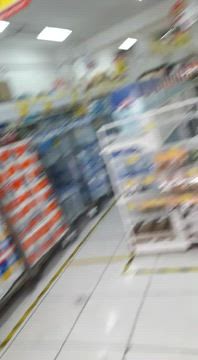The image depicts a blurred photograph taken inside a typical gas station convenience store or small shopping mart. The photograph appears to be in motion or taken without steadying the camera, contributing to its lack of focus. The floor is covered in worn-out white square tiles interspersed with darker areas and marked by yellow tape or borders running diagonally from the bottom left to the top right, including a zigzag pattern.

The scene includes an aisle filled with products displayed on shelves. On the left side of the image, there are columns of red and white striped items, possibly paper products like paper towels or toilet papers, alongside some blue packaging. Toward the right side, a white wire rack with various products can be seen, showcasing a mix of blues, yellows, and browns. 

The image also features a white ceiling illuminated by sparse, rectangular fluorescent lights, and yellow price tags are scattered throughout the products, though their exact details are indistinguishable. In summary, this blurry photograph captures a cluttered convenience store aisle with diverse products and worn-out floor tiling.